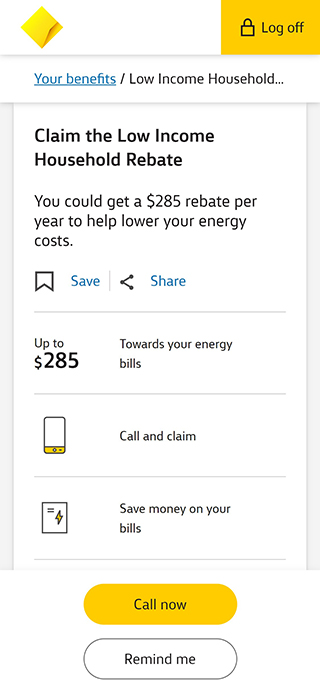The image displayed mimics a smartphone screen. At the very top left, there is a yellow to gold diamond-shaped icon. On the top right, within a gold box with black text, reads "Log Off" accompanied by a briefcase icon. Just below this, large blue text says "Your Benefits," followed by a subtitle in black that reads "Low-Income Household."

The main section of the page features prominent, bold black text on a white background that states "Claim the Low-Income Household Rebate." Below this headline, it mentions in non-bolded black text, "You could get a $285 rebate per year to help lower your energy costs."

Further down, there's detailed information about the rebate program. The text explains that this initiative offers up to $285 annually to reduce energy bills. Users have options to save or share this information.

Towards the bottom, an icon of a smartphone is displayed along with the text "Call and Claim." Adjacent to this is a small image resembling an electricity bill with the phrase "Save money on your bills." 

Centered at the bottom, there is a gold button with black lettering that says "Call Now." Next to it, outlined in light gray with a white background and black lettering is an oval button that reads "Remind Me."